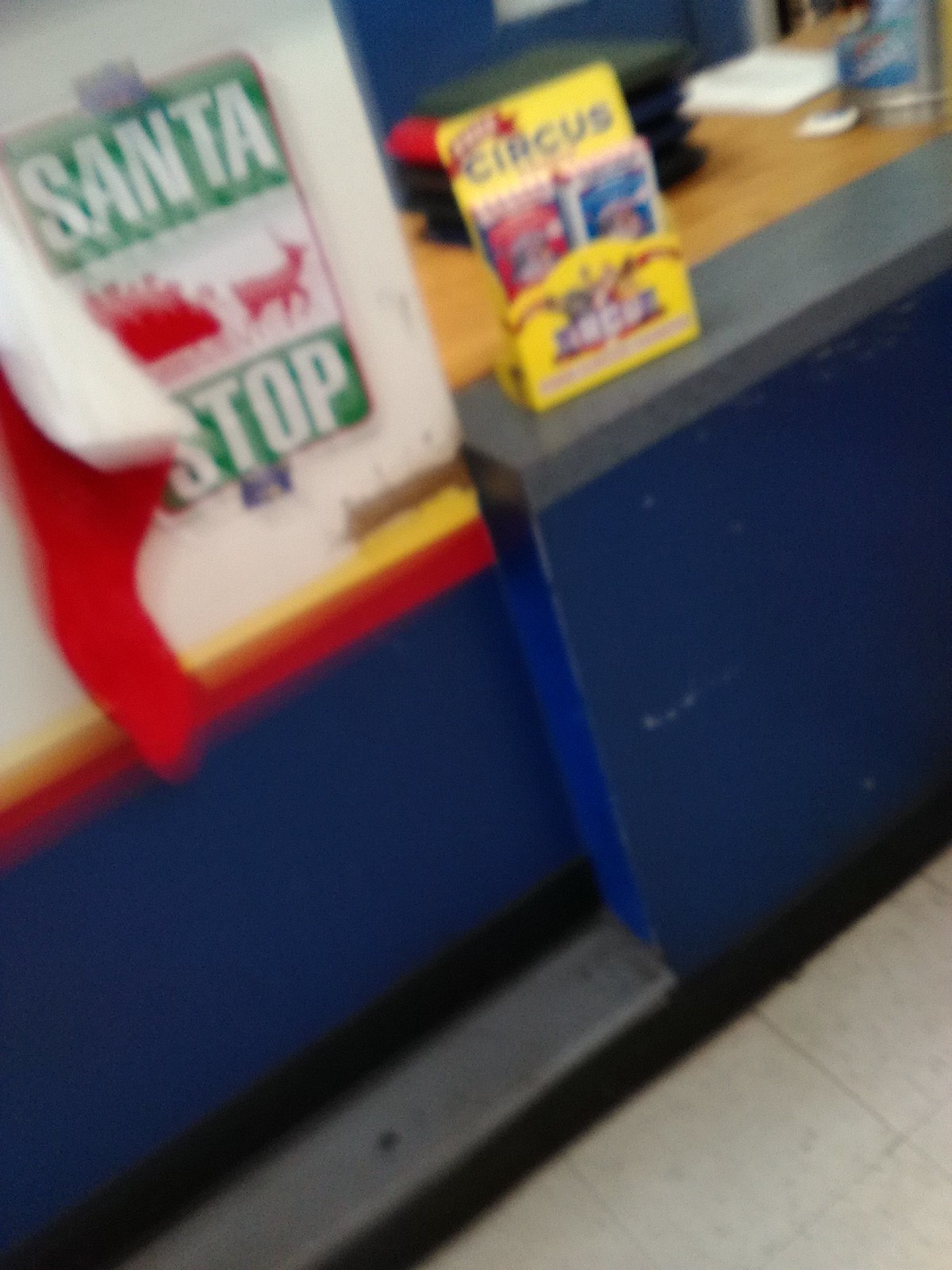This is a color photograph depicting the interior of what appears to be a retail shop or similar venue. Dominating the scene is a weathered dark blue wall that intersects with a cluttered countertop. The wall, extending toward the ceiling, features a "Santa Stop" sign prominently displayed at the forefront. Adjacent to this, a small brochure display for the circus is placed on the counter. Various objects, contributing to a slightly disorganized appearance, are scattered atop the countertop. The flooring consists of old-school linoleum tiles, appearing somewhat dingy and worn. The overall image quality is notably blurry, offering clear visibility of objects in the foreground but rendering the background indistinct. The ambiance suggests a timeworn workspace within a retail setting.